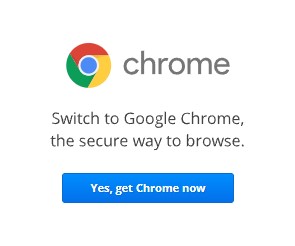The image features a prominent circle on the left side, measuring approximately 2 to 3 inches in diameter. The outer rim of the circle is segmented into three colors: red at the top, yellow in the middle, and green at the bottom. Inside this multicolored ring is a solid blue circle. 

Positioned to the right of the circle is the word "Chrome," spelled out in uppercase gray letters (C-H-R-O-M-E). Below this word, there is additional gray text that reads, "Switch to Google Chrome, the secure way to browse."

Approximately 2 inches beneath this text block is a rectangular button, measuring around 4 to 5 inches in width. The button has a blue background and contains the phrase "Yes, get Chrome now," with an uppercase 'C' in "Chrome." This is the extent of the information depicted in the image.